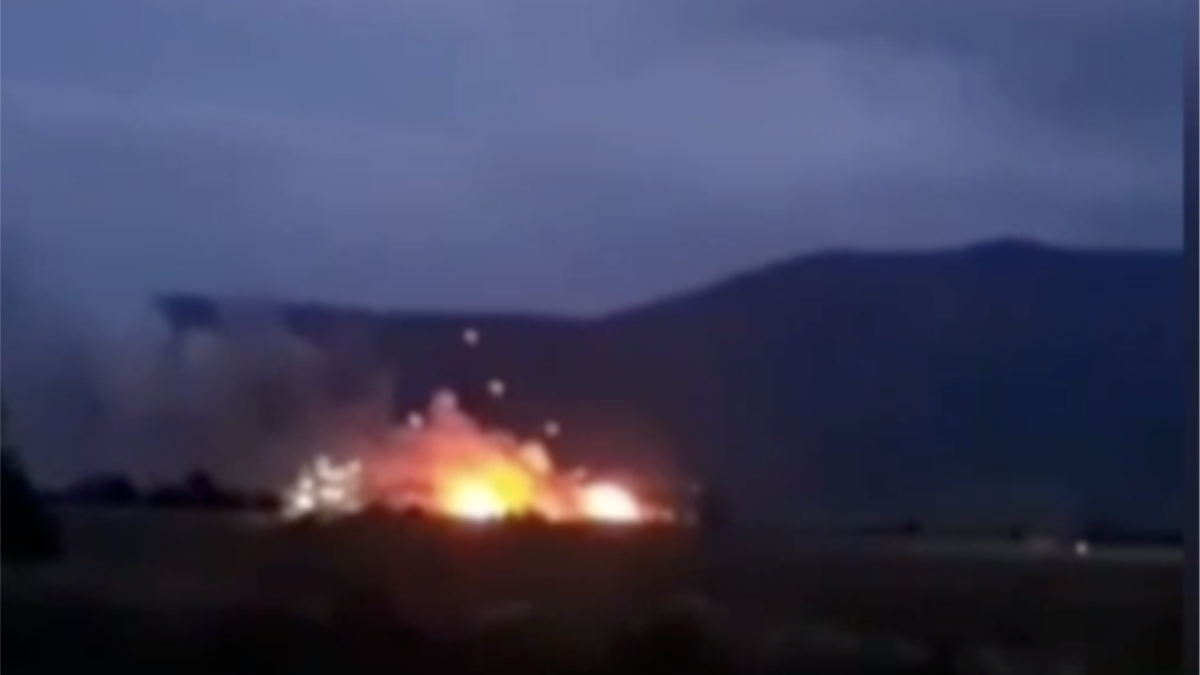The blurry nighttime image captures a dramatic explosion set against a dark, cloudy sky. In the middle of the picture, a large, fiery explosion dominates, releasing vibrant yellows, reds, and some white hot spots. The surroundings are largely indiscernible silhouettes, possibly mountains or hills, that fade into a black and bleak foreground. Scattered around the central blast are a few white dots or fragments, perhaps embers or reflecting light, intensifying the chaotic scene. Though specific details are unclear due to the blurred quality, the overall impression suggests a large-scale, powerful event such as a drone attack, volcanic eruption, or car explosion, emphasizing the sheer magnitude of the disaster and its impactful presence.